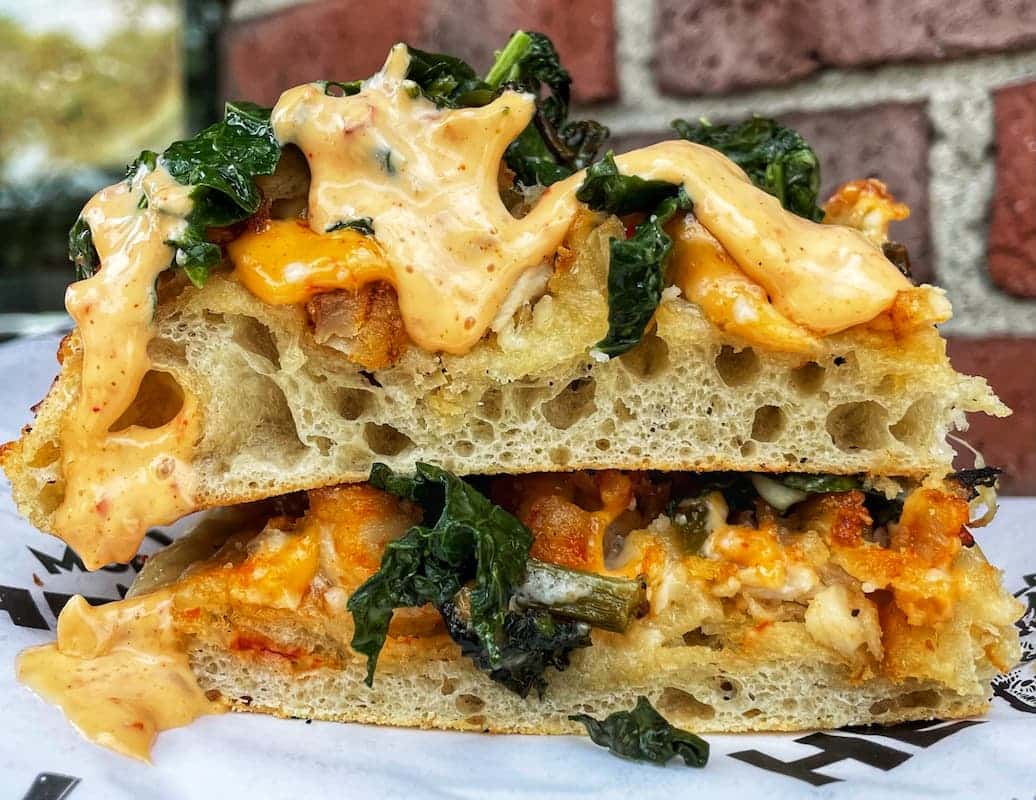This image showcases a delectable sandwich, likely photographed for a restaurant menu, set against a rustic brick wall backdrop. The sandwich consists of two pieces of light and airy focaccia or ciabatta-like bread stacked on top of one another. The bread, with visible holes that suggest its fluffy texture, cradles a mix of dark green, wilted spinach and a richly colored, possibly orange, cheese sauce that oozes enticingly over the edges. Additionally, there are hints of crispy elements within, which could be fried cheese or bacon, adding to the complexity and crunch of this appetizing creation. The entire sandwich rests on a white cloth adorned with subtle brown lettering, creating a contrasted and visually appealing presentation.